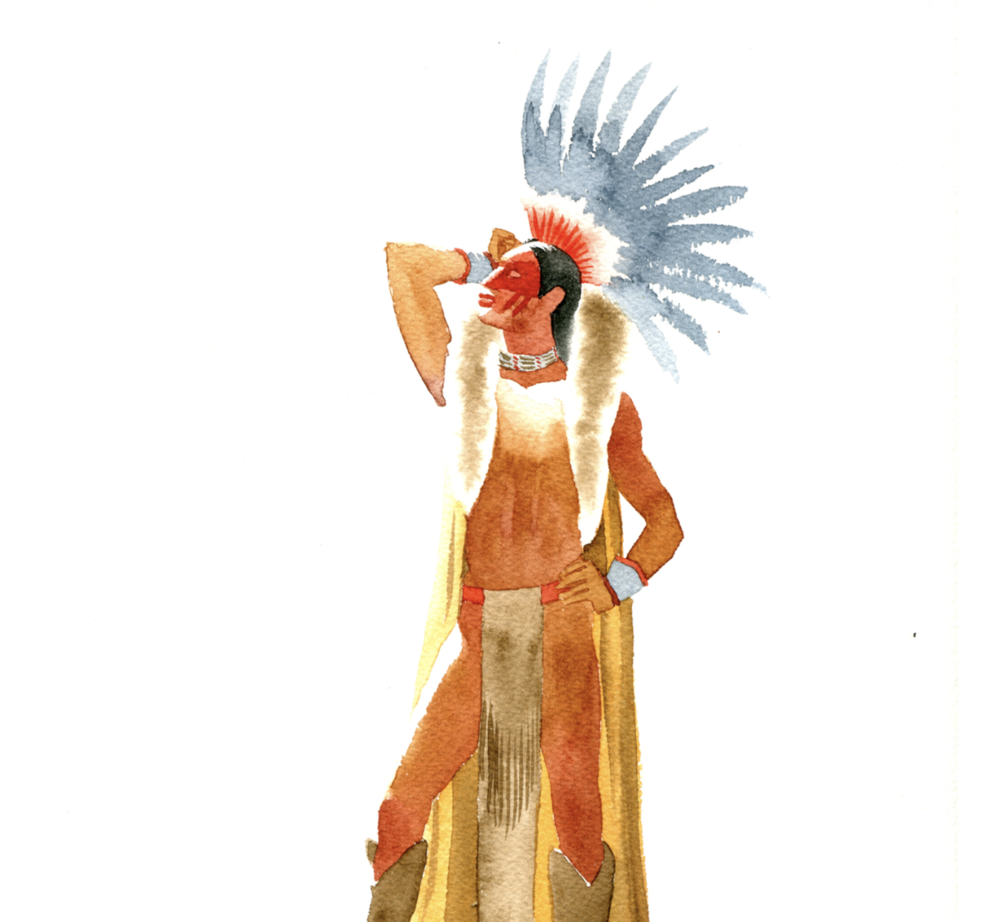This intricate watercolor painting by Kent Monkman, titled "Faint Heart 96,922," created in 2008, depicts a striking Native American man, exuding an air of both traditional and contemporary influences. The man, central to the composition which occupies the entire image, is illustrated against a stark white background. Leaning slightly back with his left hand on his hip and his right hand raised to his head, he gazes to the left, his pose both commanding and introspective.

Dressed in various traditional elements, he wears a distinctive loin cloth secured with a belt, leaving his chest and legs exposed. His dark, lengthy hair is complemented by a feather headdress featuring gradations of light blue and red. His attire includes wrist guards and a luxurious gold robe with a fur collar draped over his shoulders, reminiscent of a cape. Leather cowboy boots adorn his feet, combining elements of historical dress with modern nuances. His face, marked by red paint around the eyes that extend down his cheeks, enhances the vividness of the portrait. Around his neck, he sports a white choker, adding to his dignified appearance.

This evocative painting, not only a testament to Monkman's skill but also to his post-colonial and queer art influences, challenges and reimagines historical narratives through a modern lens.